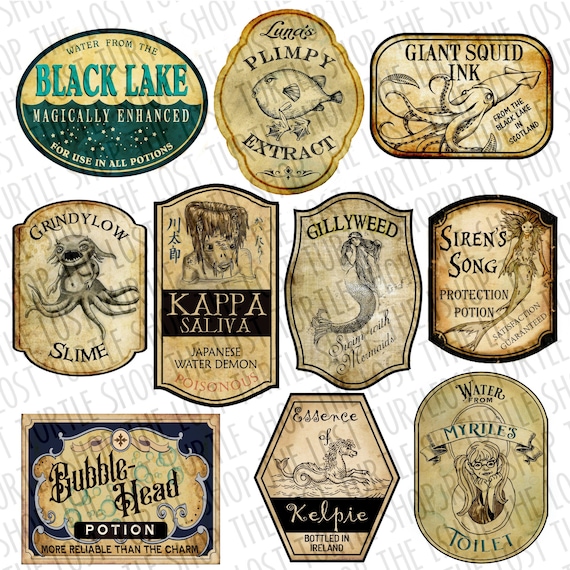This image features a collection of 10 vintage-style stickers or labels, likely intended for decoration in a whimsical, thematic setting such as a restaurant or pub with a magical or aquatic theme. The background is white with the repetitive text "The Lost Turtle Shop" diagonally across the entirety. Each sticker conveys a unique, fantastical product:

1. **Top Left**: An oval tan patch with aqua details reading "Water from the Black Lake, magically enhanced for use in all potions".
2. **Top Center**: A vertical oval with the text "Luna's Plumpy Extract" featuring an illustration of a blowfish.
3. **Top Right**: A rectangular label stating "Giant Squid Ink from the Black Lake in Scotland" with a squid drawing.
4. **Middle Left**: Another vertical oval with "Grindylow Slime" and a depiction of a fearsome sea monster.
5. **Middle Center-Left**: A vertical oval labeled "Kappa Saliva, Japanese Water Demon Poisonous" with a rendering of the mythical creature.
6. **Middle Center**: A vertical rectangle "Gillyweed, Swim with Mermaids" accompanied by a mermaid illustration.
7. **Middle Center-Right**: A rounded vertical rectangle with "Siren Song Protection Potion, Satisfaction Guaranteed" showcasing a siren drawing.
8. **Bottom Left**: A horizontal rectangle "Bubble Head Potion, More Reliable than the Charm" with blue detailing and bubbles.
9. **Bottom Center**: A diamond-shaped label reading "Essence of Kelpie, Bottled in Ireland" featuring a seahorse image.
10. **Bottom Right**: A vertical oval "Water from Myrtle's Toilet" with a picture of a toilet and Moaning Myrtle from Harry Potter.

A watermark is present across the entire image, preventing copying. The combination of imaginative elements and enchanting illustrations suggests these labels are designed for a fictitious apothecary or magical supplies store, celebrating a magical world akin to Harry Potter.